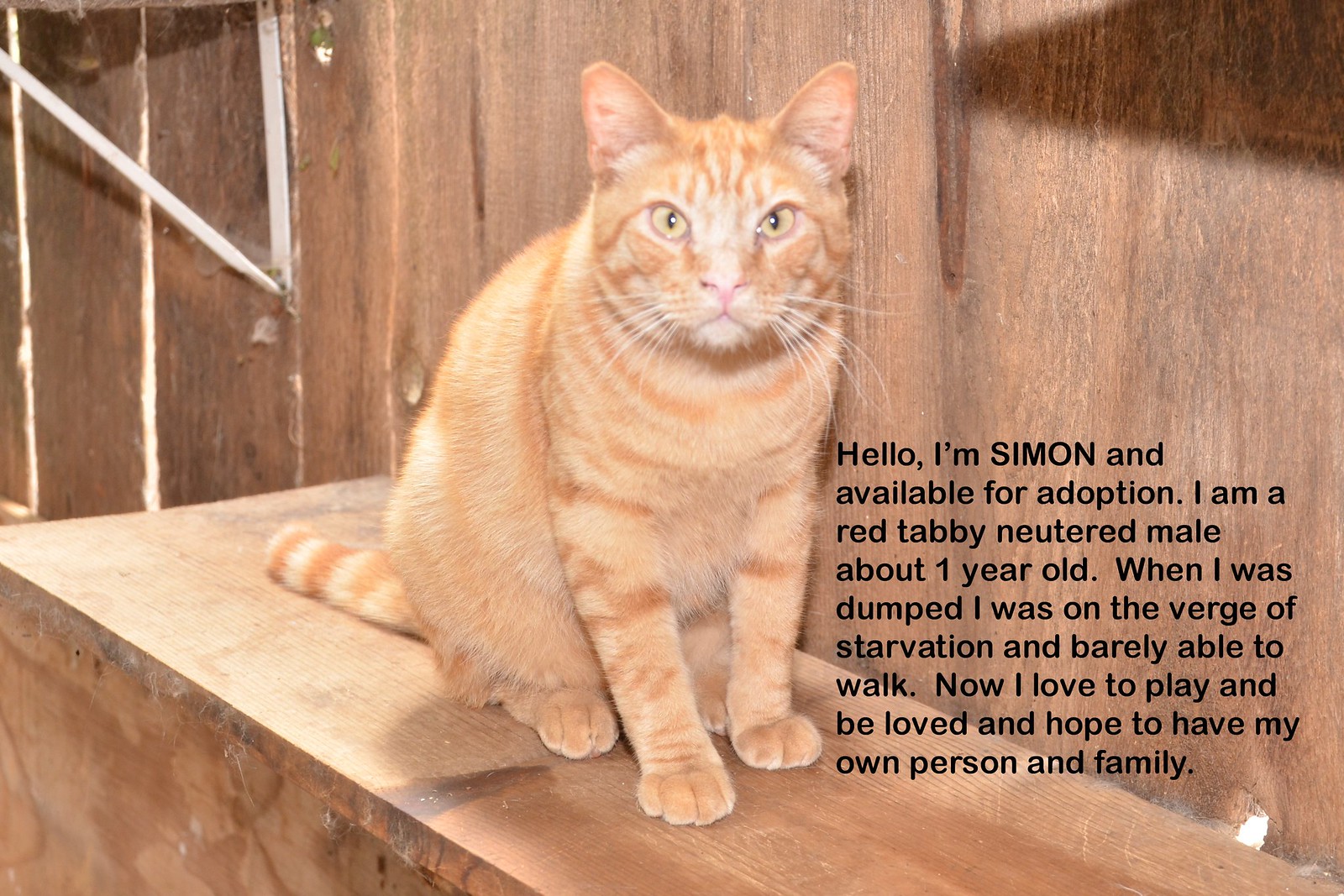This photograph features an orange-striped cat named Simon, who has light orange fur interspersed with darker orange and lighter orange stripes across his body and tail. Simon is seated on a dusty wooden plank, his front paws placed in front of him, almost half-standing as he faces the camera intently. His ears are perked up, and his yellow eyes, paired with white whiskers, give him an attentive look. The setting includes wooden walls of the same color. In the bottom right corner of the image, black text reads, "Hello, I'm Simon and available for adoption. I'm a red tabby neutered male about one year old. When I was dumped, I was on the verge of starvation and barely able to walk. Now, I love to play and be loved and hope to have my own person and family." This photograph is an advertisement from an animal shelter, seeking a loving home for Simon.